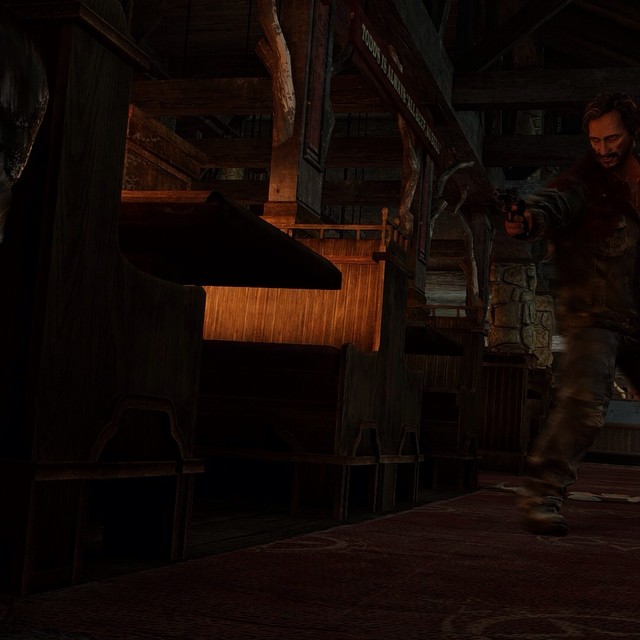The image appears to be a photograph captured in a dimly lit restaurant or eatery with a notable rustic, barn-like aesthetic. On the left side of the establishment, there are brown wooden booths with highback benches. These booths are positioned beneath wooden rafters and surrounded by brick or stone columns. The floor is carpeted with a burgundy hue. Central to the image is a man with short, dark hair, a mustache, and a beard. He is wearing a long brown or black jacket, torn jeans, and black boots, and his face conveys anger as he gazes upward while his head is tilted slightly downward. In his right hand, he holds a gun, possibly a revolver. The setting almost resembles a video game cutscene, with dark wooden structures and a few distinct, illuminated areas. Additionally, there’s white text above the different sections and bays, and a faint light emanates from one of these bays on the left. Towards the middle of the image, slightly illuminated, there is a large metallic object, possibly resembling a crane with a shovel-like attachment, and some sort of equipment with a metal circular ring hanging down. The overall ambiance is dark, with the right side of the image especially lacking light, adding a menacing and mysterious atmosphere to the scene.